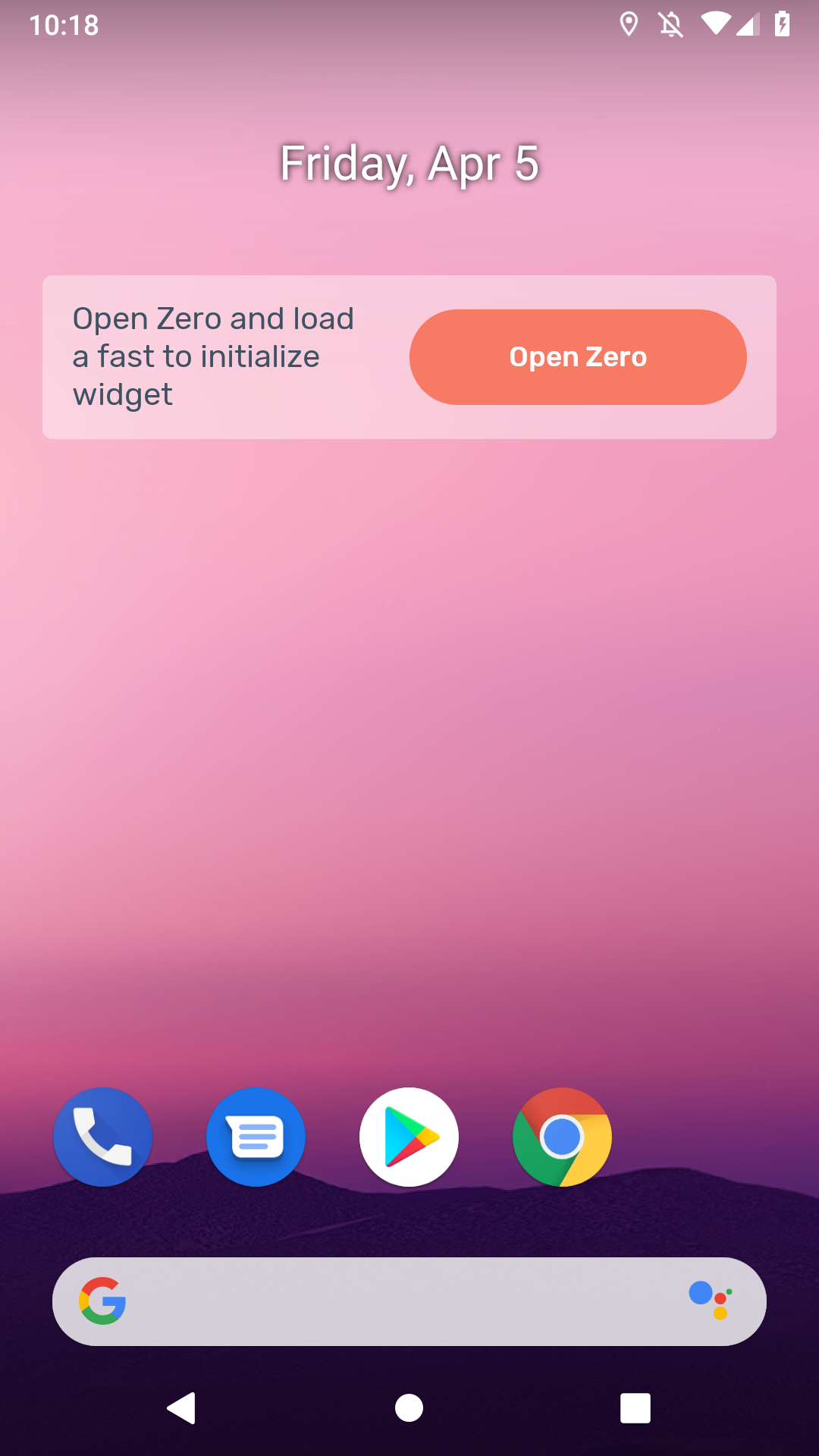A minimalistic home screen of an Android phone featuring a serene twilight-themed wallpaper. The backdrop captures a picturesque purple and pink sky, indicative of a sunset with the sun already below the horizon. Hints of light elegantly paint the sky, complemented by a subtle mountain range at the bottom, highlighting the expansive sky. 

At the bottom of the screen, a Google Assistant/search bar is prominently placed for easy access. Directly above the search bar are four essential app icons: Phone, Messages, Play Store, and Chrome, facilitating quick navigation.

A notable addition to the otherwise sparse layout is a widget with the text "Open Zero" (with a capital Z) and a somewhat cryptic message "load a fast to initialize widget," featuring a few typographical errors. There is also an actionable button labeled "Open Zero,” suggesting a function to initialize or open another widget, adding a layer of intrigue to the clean interface. This setup and the default wallpaper suggest a recently initialized phone with minimal user customizations.